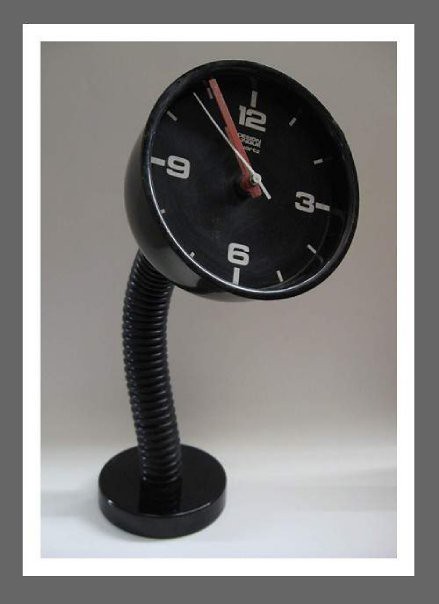This detailed photograph features an old-school style clock with a distinct design. The clock's face is circular, showcasing just four numbers: 12 at the top, 3 on the right, 6 at the bottom, and 9 on the left, all in white text. The remaining hours are marked by small white lines. The clock’s hands are prominently colored in white and red. The clock is mounted on a metal structure resembling a slinky with several horizontal ridges, allowing for flexible movement. This structure connects to a sturdy black circular base. The image background is predominantly gray with a white bottom, and minimal shadows indicate well-balanced lighting. The photo also features two borders: an outer gray border and an inner white one, enhancing the clock as the focal point.